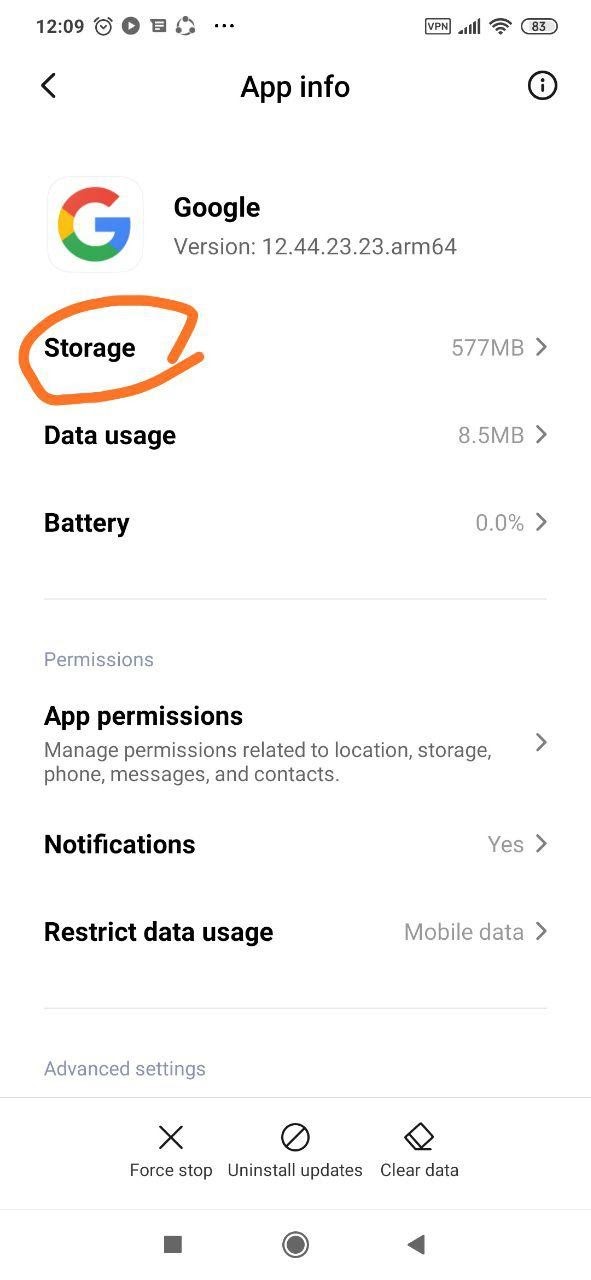**Descriptive Caption:**

This image is a screenshot from a smartphone interface, featuring a predominantly white background. At the top, "12:09" appears in black text, indicating the current time. Adjacent to the time is an alarm clock icon and a circle containing a play button. A square with text lines and another circle with surrounding dots follow next. To the far right are three horizontal dots, indicating additional options.

On the upper right side of the screen, there is a rectangular icon labeled "VPN," alongside icons showing cell signal strength, Wi-Fi signal, and an 83% battery level.

Central to the image is an arrow pointing left and the text "App Info" in larger font with a capitalized "A." Next to this text is a circle containing an information icon (an "i").

On the left side, we see the Google logo, represented by the letter "G" in distinctive multicolored segments: red, yellow, green, and blue. Beside it, "Google" is written in black text with a capital "G." Below it, the app version is specified as "version 12.44.23.23.arm64."

Beneath this, under a section titled "Storage," an orange circle highlights the app size as "577 MB," data size as "8.5 MB," and battery usage as "0.0%." 

There is a dividing line, followed by "Permissions," detailing the app's permissions with an option to "Manage permissions" for location, storage, phone, messages, and contacts. Each entry is accompanied by a right arrow.

Further down, we encounter "Notifications" set to "Yes," also with a right arrow. The "Restrict Data Usage" section mentions "Mobile data" with a right arrow. 

Lastly, under "Advanced settings," options are provided for "Force Stop" with an "X" button, accompanied by a circle with a line through it, "Uninstall updates," and a clear data function symbolized by an eraser.